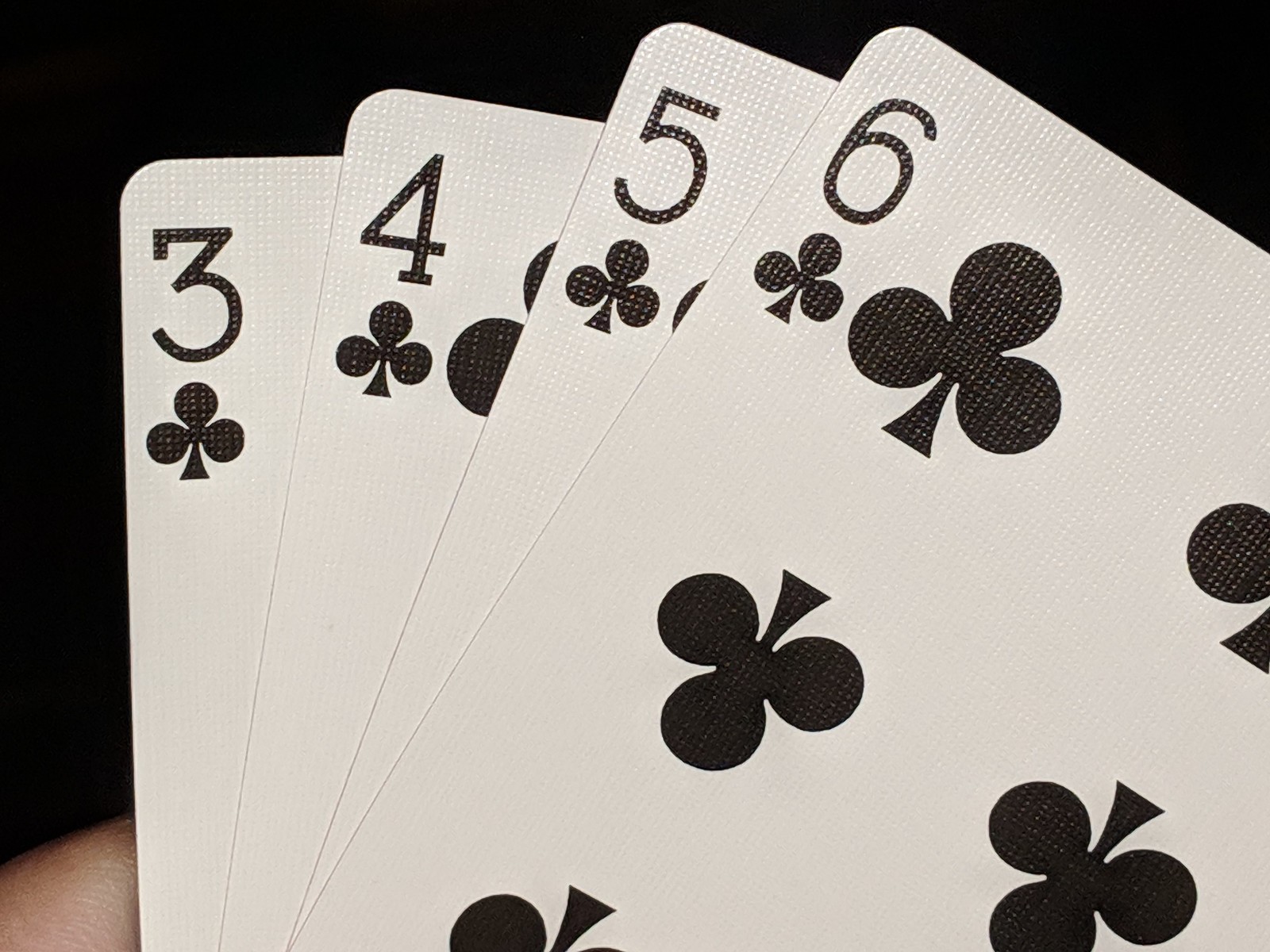In the image, four playing cards are fanned out with a predominantly black background. The top card is a Six of Clubs, displaying the six black club symbols in a pattern: the top left club is fully visible, a small part of the top right club is visible, the middle left club is completely shown, almost all of the second row right club is visible, and just a small top piece of the bottom row club can be seen. Behind the Six of Clubs is a Five of Clubs, with only the top portion including the five and one club symbol partially visible. The next card in the sequence is the Four of Clubs, mostly concealed by the Five of Clubs, with only a glimpse of one club symbol emerging from beneath the five. The last card, the Three of Clubs, is almost entirely hidden under the preceding cards, revealing just the numeral three and a partial club symbol. A hand appears in the bottom left corner, holding the cards, and the skin tone of the hand is Caucasian.